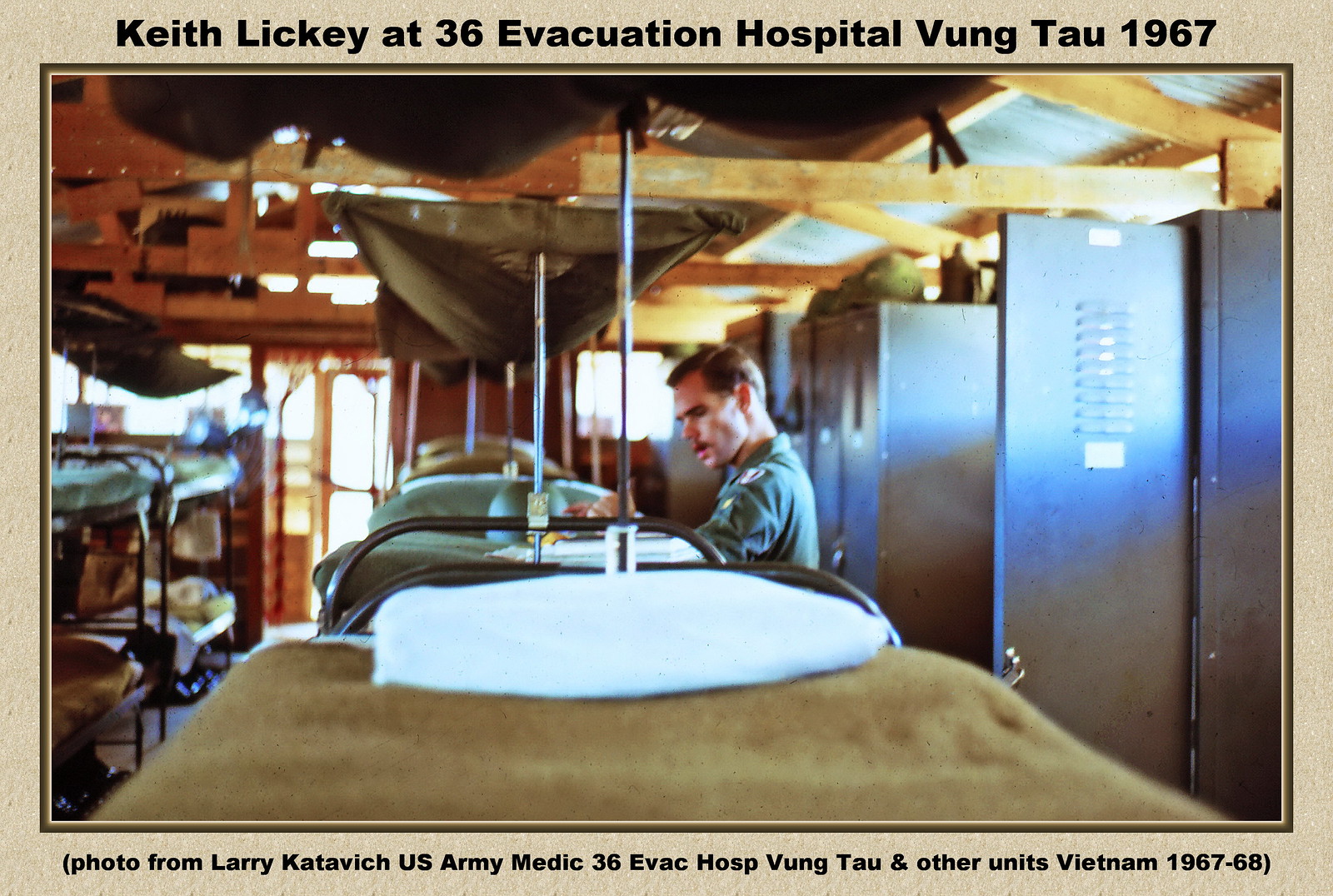The photograph captures a serious and somber moment within a large room of the 36th Evacuation Hospital in Vung Tau, Vietnam, circa 1967. The image prominently features a man with a mustache, dressed in a green uniform, standing to the right of a row of bunk bed cots and open gray lockers. These lockers are aligned against the background where additional cots and the wooden support beams of the ceiling are visible. The scene is tinged with colors ranging from different shades of brown and green to gray, white, and black, giving the impression of an environment marked by the austerity of military life. Above the man, text in black reads "Keith Lickey at 36 Evacuation Hospital, Vung Tau, 1967," while the bottom of the photograph notes "Photo from Larry Katovich, US Army medic, 36 Evac Hospital, Vung Tau, and other units, Vietnam, 1967-68." The photograph is bordered in brown and set against a light tan background, further enhancing its historical and serious ambiance.